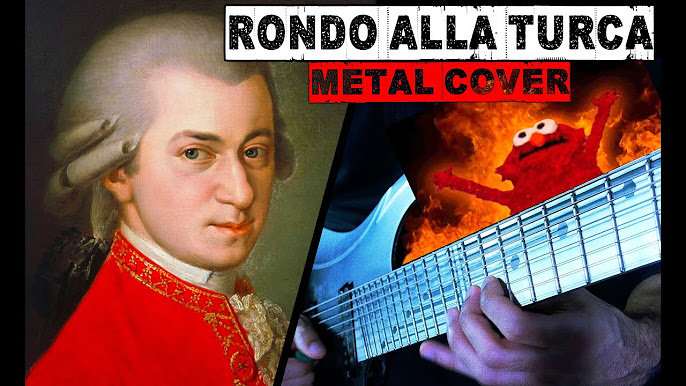The image appears to be a striking and imaginative album cover for "Rondo alla Turca Metal Cover." On the left side, it features an 18th-century figure reminiscent of a young George Washington or Mozart. This figure is adorned in a red coat with high-collar white shirts, a powdered wig with curls, and a gold bow tied across his chest. On the right side, there is a depiction of close-up human hands playing an electric guitar, with the body of the guitar partially obscured by a black t-shirt emblazoned with an image of Elmo, seemingly signaling a wild and unconventional "Crazy Elmo" persona. The background shows dark contrast with flames, adding a dramatic and intense atmosphere to the composition.